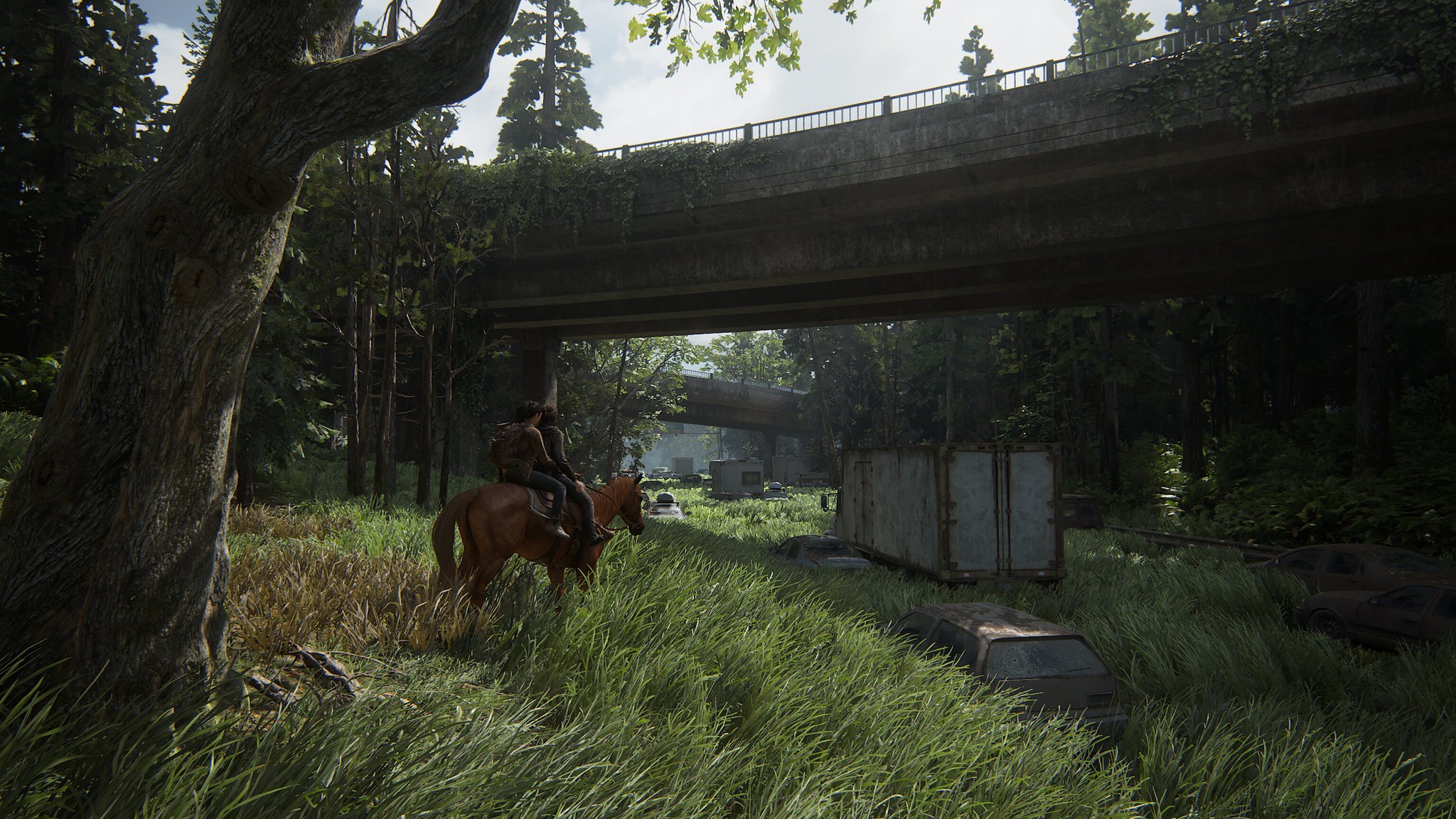This image, which evokes a mildly post-apocalyptic atmosphere, captures two people on a brown horse, facing to the right, under a stone, vehicle bridge. Surrounded by overgrown flora, the tall, lush grass encroaches on abandoned vehicles, including a semi-trailer and rusted cars, suggesting a once-busy road now reclaimed by nature. The background features a second bridge that seems to mirror the first, heading in a different direction amidst a forest of tall pine trees. To the left of the image, a large, knobby, gray tree trunk with small leaves stands prominently. The sunlight casts a serene yet eerie glow over the scene, making it difficult to discern if the image is a photograph or an artist's detailed rendering. The couple on the horse seems to be contemplating the surreal, abandoned landscape before them.